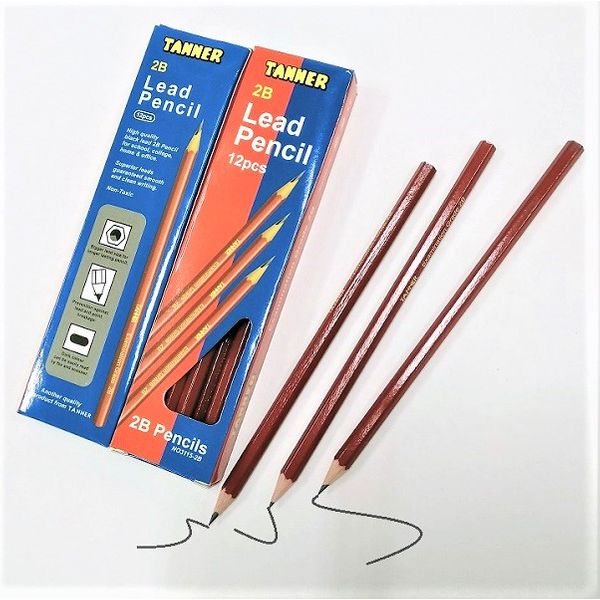This nostalgic product image, reminiscent of 70s or 80s design, features Tanner 2B lead pencils against a flat white background. Toward the left, two rectangular boxes of pencils are positioned side by side: the left box is blue and displayed face down, showing detailed product information including "Tanner 2B Lead Pencil," "high quality," "black lead," and "smooth and clean writing," with a depiction of a single pencil. The right box, blue and orange, is face up, displaying "Tanner 2B Lead Pencil, 12 pieces" with three pencil images and a small plastic cutout revealing the brown pencils inside. At the bottom, additional labeling reads "2B Pencils" and includes the model number "03115-2B." To the right of these boxes lie three sharp, unused pencils exhibiting brown-painted wood, each having drawn a black squiggle line on the white surface beneath them.